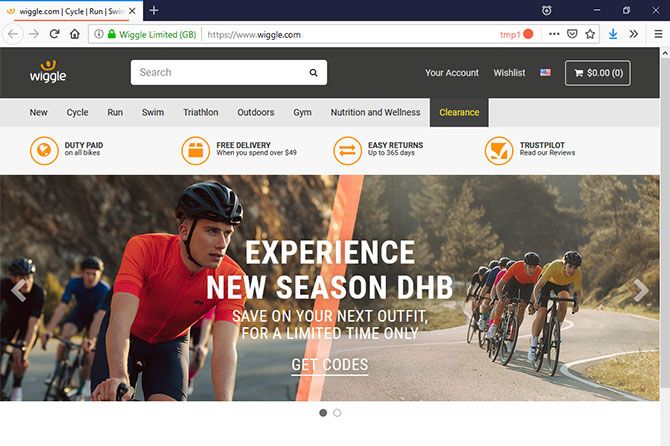In the screenshot from wiggle.com displayed in a web browser, the URL bar prominently shows "https://www.wiggle.com." The browser appears to have only one tab open, and the title of the tab reads "Wiggle | Cycle, Run, Swim" before it gets cut off. A recording indicator, represented by a red circle labeled "tmp1," is visible to the right. 

Below the top taskbar, various UI elements of the Wiggle website are detailed. The search bar is located on the right, followed by options for "Your Account," "Wishlist," an American flag symbolizing language preferences, and a shopping cart icon showing zero items with a total value of $0. 

Navigational links are prominently displayed, including categories such as "New," "Cycle," "Run," "Swim," "Triathlon," "Outdoor Gym," "Nutrition," "Wellness," and "Clearance," with the "Clearance" tab currently selected. The "Clearance" section reveals four promotional options: "Duty Paid on All Bikes," "Free Delivery When You Spend $109," "Easy Returns Up to 365 Days," and "Trustpilot Radar Reviews."

A large, full-width rectangular banner image showing cyclists riding on a road serves as the main visual element. Overlaying the image is the text, "Experience New Season DHB," with a subheading, "Save on your next outfit for a limited time only." A link located beneath this text invites users to "Get Codes."